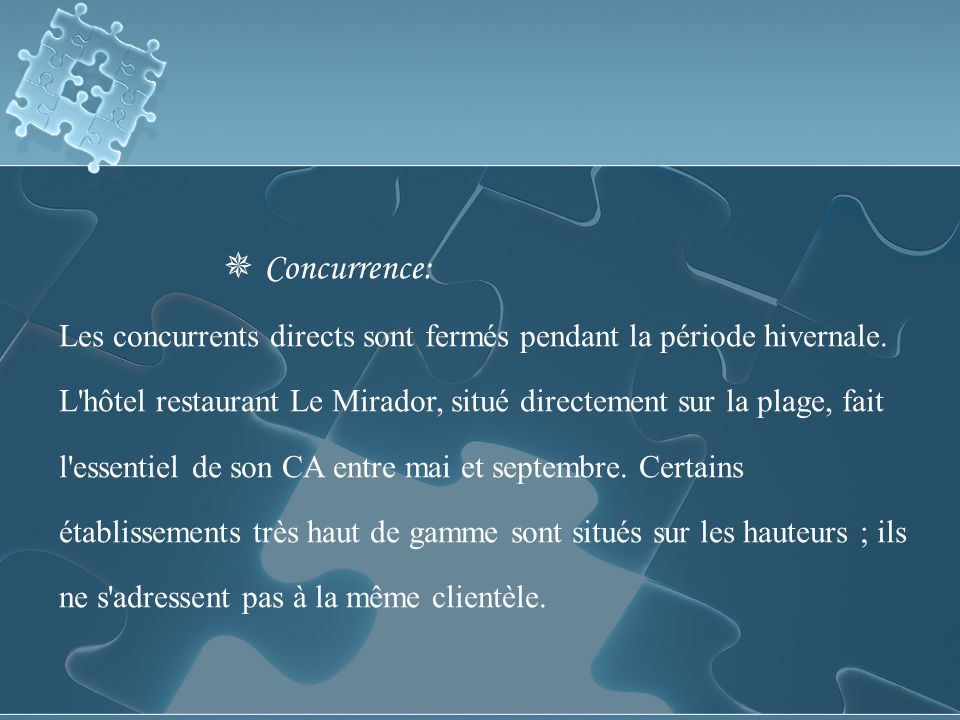The image features a blue background composed of interlocking puzzle piece designs. The upper part of the background is light blue, resembling a clear sky. Positioned in the upper left corner, there is a rotated square puzzle with a central piece missing, comprising several interconnected white puzzle pieces. The lower part of the background maintains the puzzle motif, with dark blue pieces outlined in white.

In the bottom center of the image, a single grayish puzzle piece is highlighted. This piece contains the word "Concurrence" written in white text, slightly off-center to the left with a star beside it. Below, five lines of text are displayed in French, beginning with "LES Concurrence" and concluding with the word "clientele." The exact phrases in this text include "less concurrence" followed by words and phrases that are difficult to fully decipher but suggest an array of French terms related to competition and clientele.